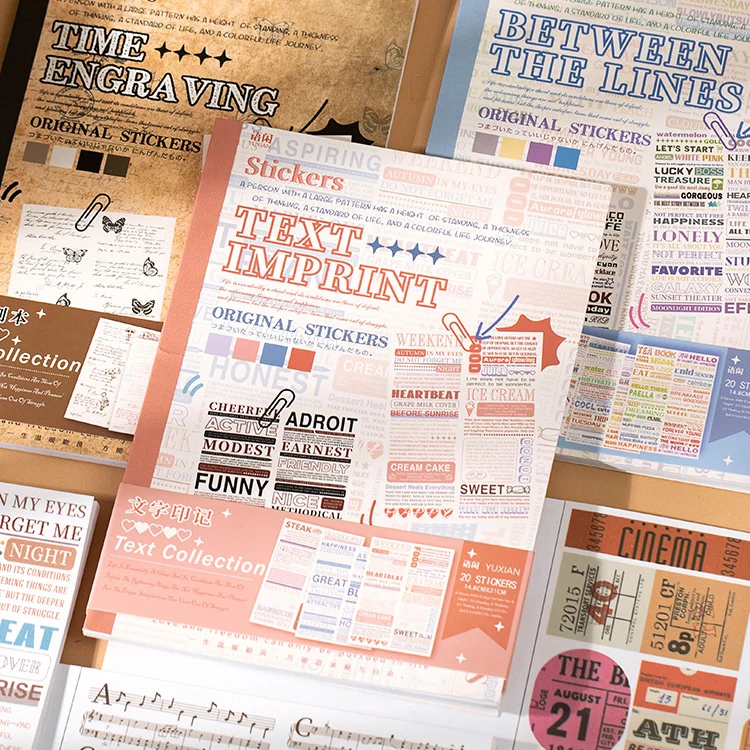This vibrant Etsy shop graphic showcases a collection of beautifully designed scrapbooking books, each accented with distinctive original stickers. The books are artfully layered, creating a visually appealing composition. 

In the top right, the first book titled "Time Engraving" features an enchanting cover adorned with intricate butterfly stamps. Next to it, "Between the Line" offers a rich assortment of word stickers like "Lucky Treasure," "Gorgeous," "Happiness," "Not Perfect," and "Galaxy," each in varied colors, encapsulating a wide range of sentiments. This book includes 20 pages of stickers.

Prominently placed at the center, the book "Text Imprint – Original Stickers" showcases words such as "Heartbeat," "Grape," "Milk," "Adroit," and "Methodical," providing an eclectic mix for creative expression.

Lower in the arrangement, one book displays sheet music, adding a musical charm to the collection. Another book, on the bottom left, appears to be themed around movies and receipts, perfect for scrapbooking travel memories or cinema experiences.

This detailed assortment of scrapbooking books and stickers offers endless possibilities for personalizing and enhancing special projects.